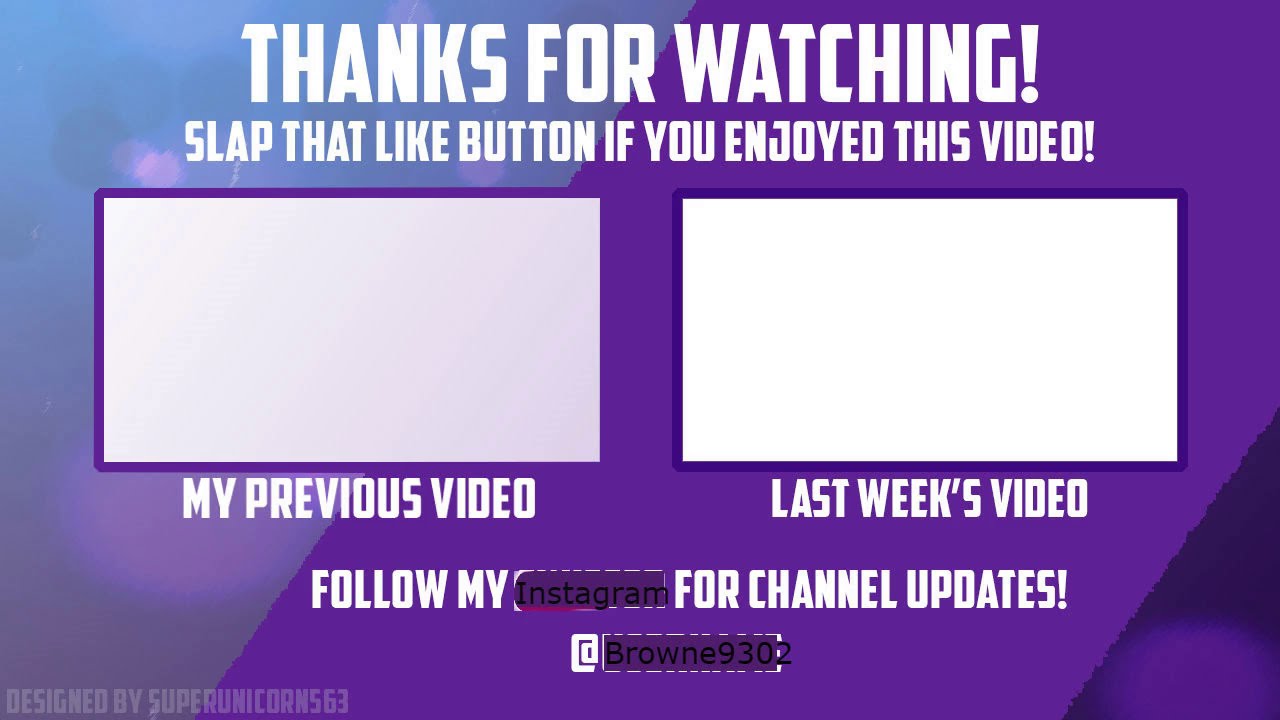The image showcases a visually striking end panel typically seen at the conclusion of a video. The background features a sophisticated pattern of diagonal stripes transitioning from blue on the left to purple on the right, culminating in a deep, dark blue-purple in the bottom right corner. At the top-center, bold white font declares, “Thanks for watching!” followed by a smaller, yet prominent, “Slap that like button if you enjoyed this video.”

Below this text, two side-by-side rectangles offer pathways to more content: the left rectangle, subtly tinged with an off-white purple hue, invites viewers with the label “my previous video,” while the right rectangle, a pure white, suggests “last week's video.” 

Further down, viewers are encouraged to engage through social media, with the instruction, “Follow my Instagram for channel updates, @Browne9302," where "Browne" is distinctly spelled out as B-R-O-W-N-E. The lower-left corner discreetly credits the designer, with the faint script reading "designed by superunicorn563."